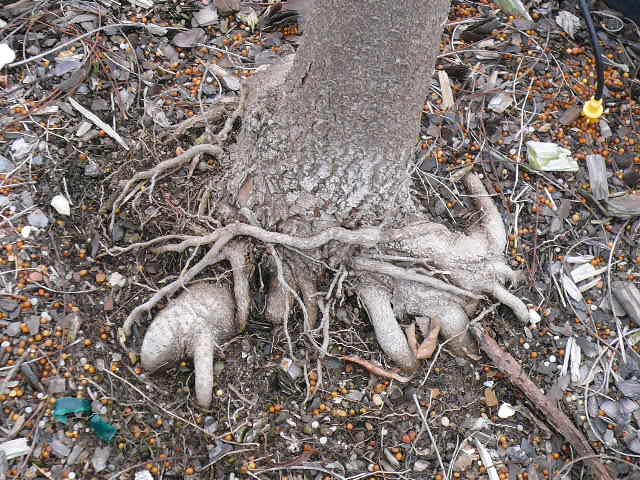This detailed color photograph, in landscape orientation, depicts a large, uprooted tree centrally framed in an outdoor setting. The trunk of the tree is a medium gray color, while the thick, gnarly roots are lighter, featuring various random shapes and configurations that have risen above the ground level. The scene around the tree roots is a mixture of dirt, pebbles, sticks, and some debris, including a smashed package and a broken bottle, highlighting a sense of neglect. Scattered on the ground are orange berries that add a touch of color to the otherwise neutral-toned environment. On the upper right side of the image, there's a black extension cord with a distinctive yellow plug-in cap that dangles downward, contributing an element of human presence to the natural chaos. The photograph is characterized by its realistic and representational style, emphasizing the juxtaposition between nature and human activities.